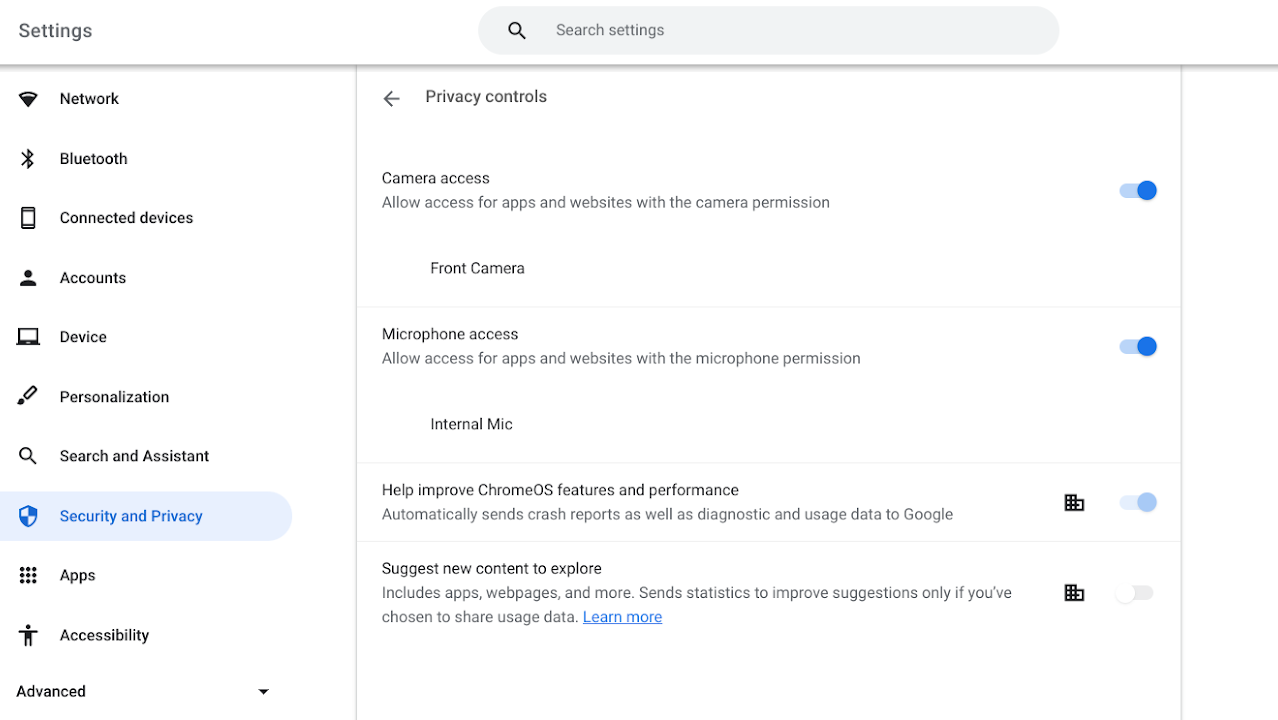This image features a web page showcasing the settings interface of a Chrome OS system. On the left-hand side, there is a vertical menu in black text listing various categories: "Network," "Bluetooth," "Connected Devices," "Accounts," "Device," "Personalization," "Search and Assistant," "Security & Privacy" (with a blue background color), "Apps," "Accessibility," and "Advanced."

At the top of the web page, a gray search bar labeled "Search Settings" is displayed. The main section of the page is headed "Privacy Controls," with a left-pointing arrow next to it. The page provides settings for "Camera Access," which is currently enabled, indicated by a blue circular slider. Below this setting, the text reads, "Allow access for apps and websites with the camera permission," followed by an additional label, "Front Camera."

Similarly, "Microphone Access" is enabled, as evidenced by another blue slider. The description here states, "Allow access for apps and websites with the microphone permission," and is followed by "Internal Mic."

Additionally, the section includes an option labeled, "Help Improve Chrome OS Features and Performance," which is not enabled; this is indicated by a black bar with two boxes – one filled with black squares, and one plain, forming an "L" shape, and displayed in light blue. This setting would automatically send crash reports and diagnostic and usage data to Google if turned on.

Lastly, the "Suggest New Content" option is also not enabled, as indicated by the absence of a blue slider. The description here mentions exploring and learning more about new content, but this option remains turned off.

Overall, the image gives a thorough overview of Chrome OS privacy controls and settings related to camera and microphone access, as well as system performance and new content suggestions.